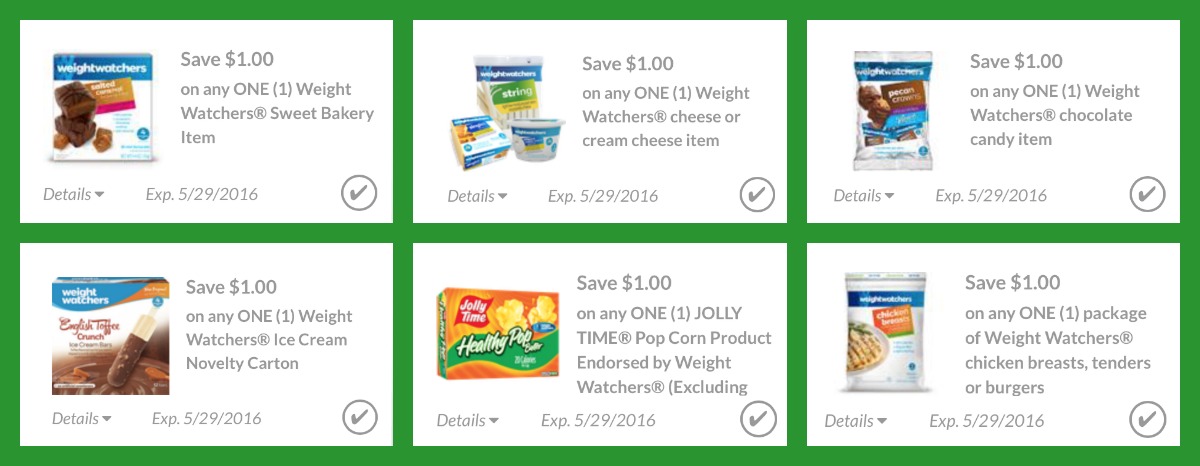The image is a rectangular, horizontally-oriented graphic divided into six individual rectangular sections, all separated by green lines—one horizontal and two vertical—forming a green-bordered grid. Each section represents a distinct grocery store coupon. The content of each coupon includes an image of the product, the savings amount ("Save $1"), a brief product description, and additional coupon details accessible via a drop-down menu. An expiration date is noted for each coupon, and a circled check mark appears in the lower-right corner of each section. 

- **First Coupon:** Save $1 on any one Weight Watchers sweet bakery item featuring an image of chocolate brownies.
- **Second Coupon:** Save $1 on any one Weight Watchers cheese or cream cheese item.
- **Third Coupon:** Save $1 on any one Weight Watchers chocolate candy item.
- **Fourth Coupon:** Save $1 on any one Weight Watchers ice cream novelty carton.
- **Fifth Coupon:** Save $1 on any one Jolly Time popcorn product.
- **Sixth Coupon:** Save $1 on any one package of Weight Watchers chicken breast tenders or burgers.

Each box is designed to clearly present the offer, making it easy for the consumer to identify the savings and the specific Weight Watchers or Jolly Time product associated with the coupon.